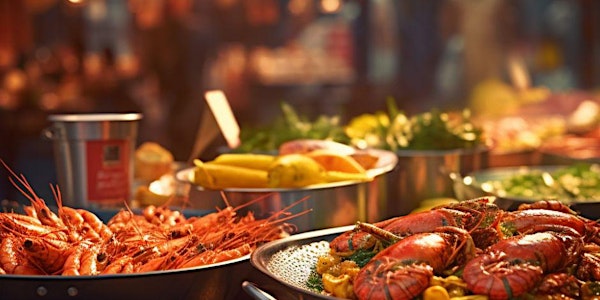This image captures a bustling seafood feast, likely set in a restaurant's banquet area. The table is laden with an array of dishes in various plates, bowls, and large stainless steel pots and pans. Central to the spectacle are bright red crawfish and lobsters, nestled among pots of vibrant green vegetables, including leafy greens and squash, as well as yellow corn and plantains. The food is artfully arranged, creating a colorful mosaic of reds, greens, yellows, and other hues that highlight the freshness and variety of the seafood and vegetables. The background, although blurry, reveals a lively ambiance with lights, tables, and people seated, suggesting a busy and enthusiastic dining environment. The scene exudes the atmosphere of a grand seafood buffet, with an abundant and visually appealing display of dishes ready for serving.